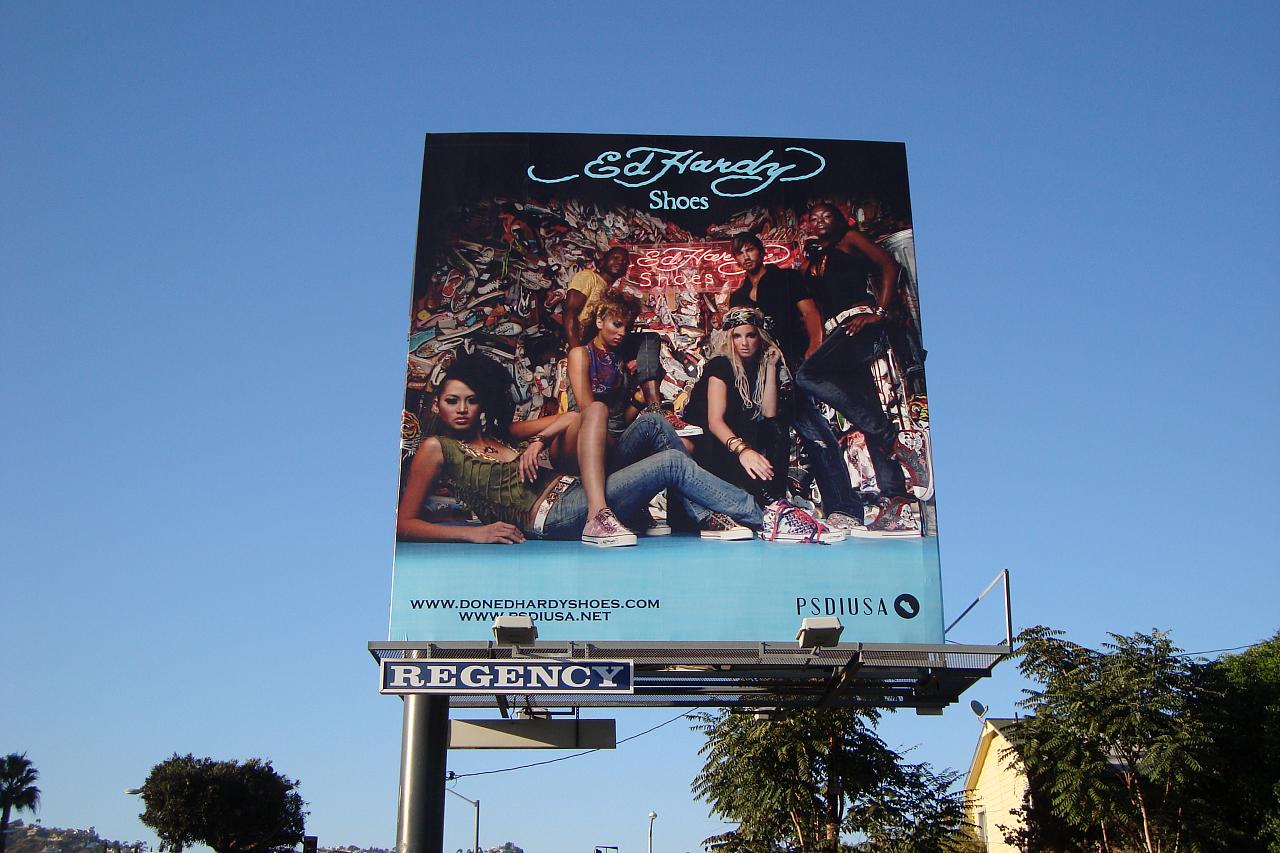The image showcases a large, square-shaped billboard prominently featuring an advertisement for Ed Hardy Shoes. At the top of the billboard, the brand name "Ed Hardy Shoes" is artistically rendered in light blue scroll letters against a black background. The central visual theme depicts six young individuals of diverse ethnic backgrounds, relaxed and exuding casual confidence. 

The group includes two African American women, an African American man, a Caucasian woman, a darker-skinned man, and another African American woman who stands out by standing up while the others are reclining. Each person sports a unique style, with various types of jeans ranging from dark to light wash. Their tops are summery and casual, featuring short sleeves, spaghetti straps, and open button-ups. The men wear t-shirts, one in bright yellow and the other in an open button-down shirt.

Behind this lively group, graffiti-styled colors provide an artistic backdrop, and the name "Ed Hardy Shoes" appears again in striking red, neon-like letters. The footwear on display includes a variety of casual tennis shoes, or court shoes, featuring designs such as animal prints, metallic finishes, and high-top styles.

At the bottom of the billboard, a blue banner displays a website URL, though part of the URL is partially obscured by a light fixture integrated into the billboard's platform, making it unreadable. The visible text is "www.donedhardyshoes.com." The billboard is identified as belonging to the company "Regency," noted in white letters on a blue background.

The billboard stands against a bright, clear blue sky, mounted on a sturdy, heavy post. Surrounding the structure are natural elements including trees on both sides and a light exposure of a yellow house roof with a satellite dish. In the distant background, a few street lights can also be spotted.